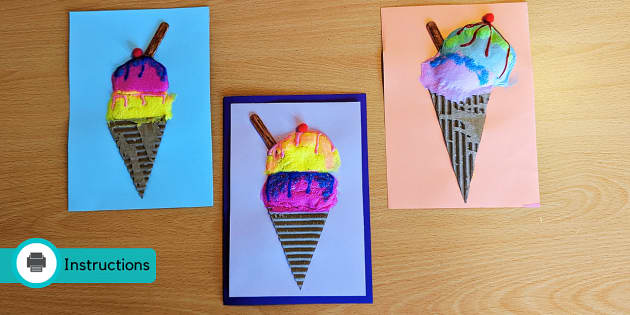The photograph depicts three meticulously crafted paper artworks displayed on a light wooden table. Each piece features an ice cream cone created from vibrant construction paper, all arranged neatly to form a striking promotional banner encouraging the art of paper crafting. In the bottom left corner, overlaid on the image, a blue banner with a white printer icon and black text reads "instructions."

The top left artwork showcases a blue background with a vibrant ice cream cone boasting a colorful 3D appearance, adorned with bright pink and yellow scoops, crowned by a cherry, and accented with a stick resembling a cinnamon stick.

Centrally, the second piece is set on a purple sheet with a blue border. This ice cream cone contrasts with deep purple and blue scoops on the bottom, and layers of red, pink, and yellow scoops piled high, again topped with a cherry and a decorative stick.

On the right, the final craft is displayed on peach-colored construction paper. This ice cream cone features similar colorful mounds of ice cream, keeping the theme of a cherry on top and a stick decoration. The combined use of bold colors like bright pink, yellow, deep purple, and blue across the cones creates a visually cohesive and appealing display, perfect for grabbing attention and inspiring creativity.